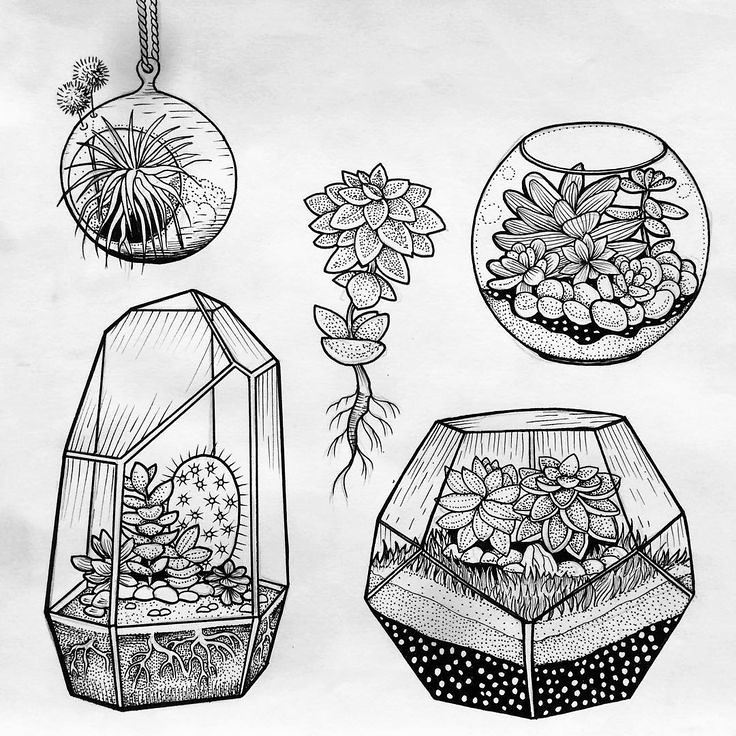This image is a detailed black and white sketch on a light gray background, showcasing various plant arrangements within different terrarium-like containers. In the top left corner, there is an orb-shaped pendant suspended by a chain, containing intricate drawings of spiky plants and air plants. Beneath this, a larger terrarium features a cactus enclosed in a glass container, with its roots visibly extending into the soil.

At the center of the image lies a standalone, leafy flower with buds along its stem, extending downwards to exposed roots. This serves as a natural divider between the terrariums.

To the right, in the upper section, a small bowl holds a variety of plants, with layers of rocks and soil visible but no roots. Directly below, a hexagonal glass enclosure contains succulents and some grass, with noticeable sediment and white dots in the soil, suggesting varied plant textures.

In the bottom left, an elaborate crystal-shaped terrarium includes succulents and a cactus, with its roots embedded in a drier soil mixture enhanced by small round rocks.

Each terrarium blends art and nature, illustrating potential designs for plant holders, emphasizing cacti, succulents, and air plants in visually striking containers.